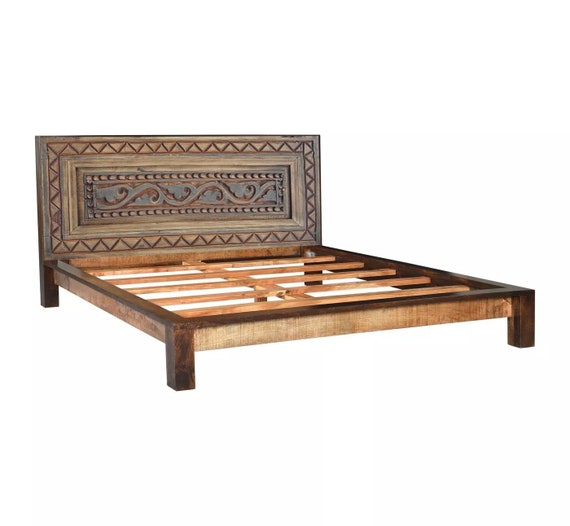This image depicts a meticulously crafted king-size bed made entirely of wood, set against a blank backdrop. The bed frame is relatively low in height but broad in width, and it is supported by blocky, chunky wooden legs that exude a sense of sturdiness. The decorative headboard steals attention with its intricate carvings. It features a triangular border, within which lies an ornate inlay panel adorned with graceful, flowing designs of leaves and vines, all intricately carved. The entire bed is a rich brown color, showcasing varying shades of wood; the inlay with the leaves is a darker hue compared to the surrounding rectangular frame. The bed frame is equipped with five supportive slats.